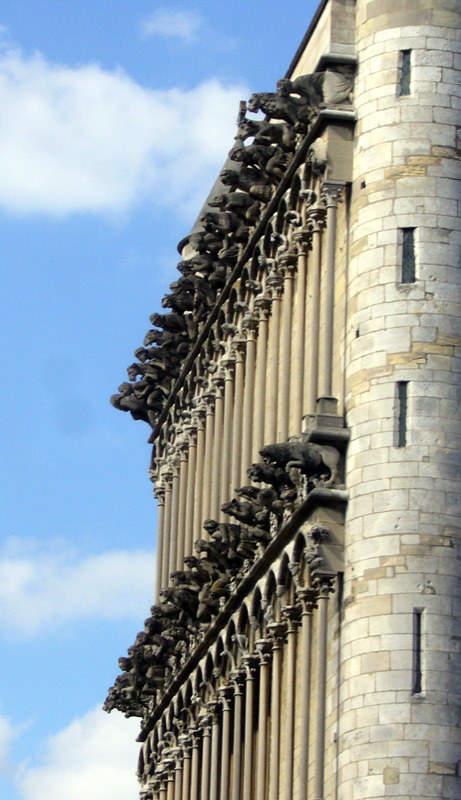The image captures the side of a castle-like building in a color photograph taken in portrait mode. The scene is set against a vibrant blue sky dotted with white, billowy clouds. Dominating the right side of the frame is a cylindrical tower or turret made of light grey stone with diagonal streaks of light brown, mimicking the contour of a spiraling stairwell inside. The turret features narrow, slit-like windows that accentuate its curved architecture. Extending from the tower towards the left is a row of stone columns with arches, creating a ribbed colonnade. Each column is topped with ornate sculptures resembling gargoyles, grouped in two dense rows. These dark grey gargoyles appear intricately detailed and highly clustered, adding a gothic flair to the overall scene. The comprehensive architectural elements and the multitude of gargoyles give the building a formidable yet captivating presence, accentuated by the serene sky above.